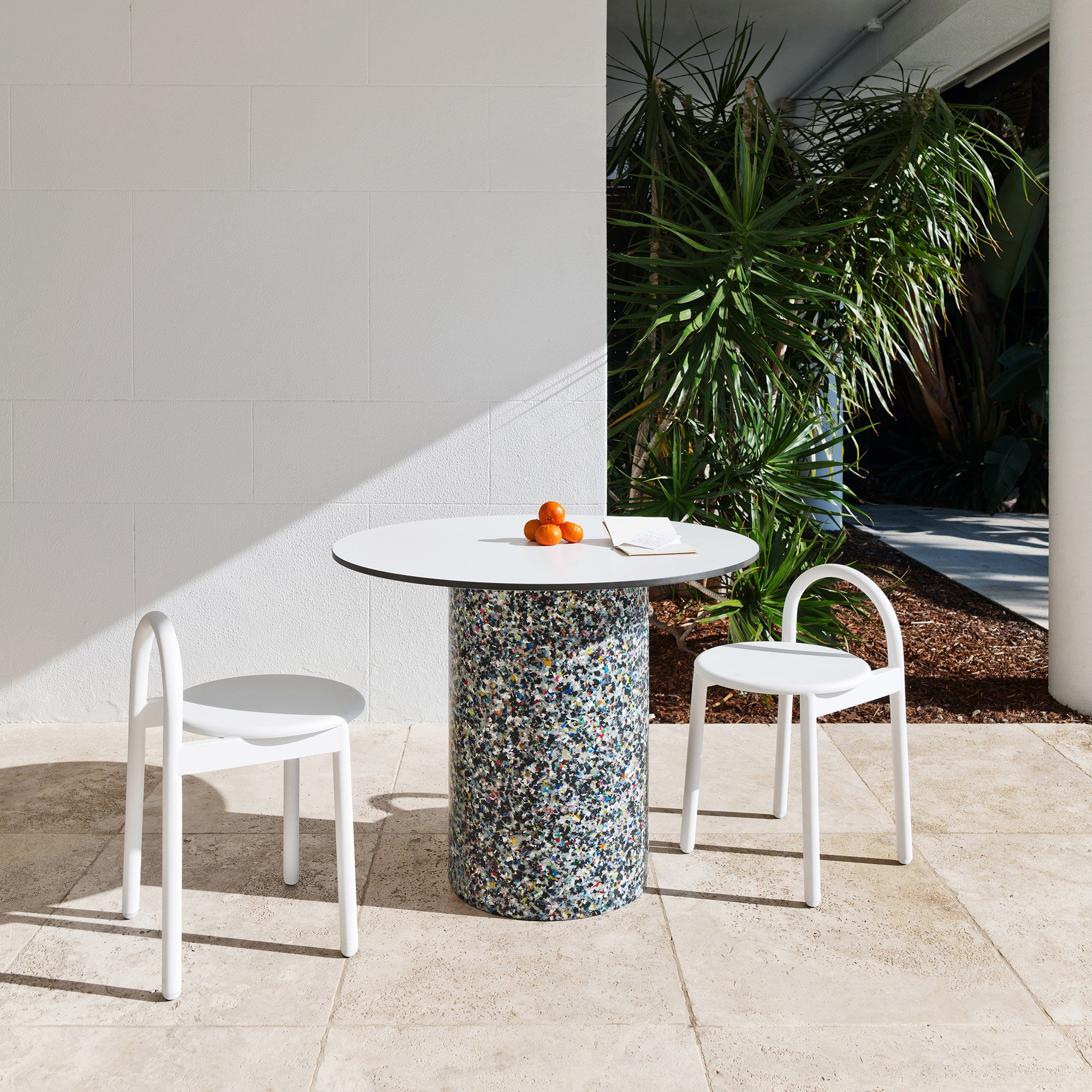The image features a contemporary outdoor seating area adjacent to a building. The setting is decorated with large, tan tiles paving the ground. The focal point is a modern, round, white table with a unique cylindrical base composed of a colorful aggregate of various stones, resembling a fish tank's mosaic. Atop the table rests a neat arrangement of four oranges and an open notebook.

Flanking the table are two minimalist, low-backed white chairs with round seats. Behind the seating area, a white wall extends with a white pillar visible on the right, connecting to a roof. Near the seating area, a square mulch bed hosts tall, fern-like tropical plants, suggesting a warm climate akin to Florida or California. Extending from this area is a walkway that further underscores the inviting outdoor atmosphere. The overall scene is bathed in bright light, with a hint of shadow in one corner, capturing a tranquil, sunlit moment.